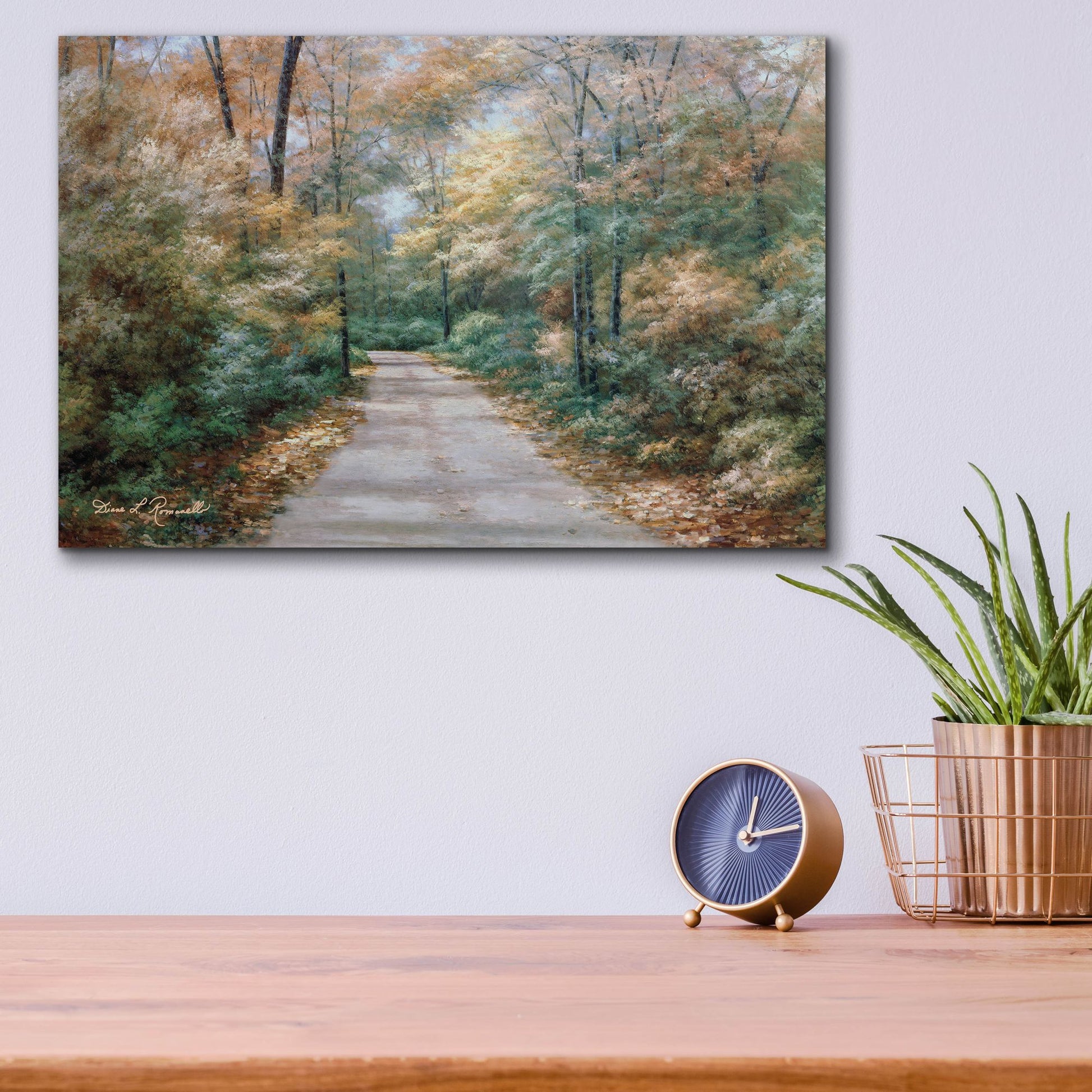The photograph showcases a beautifully detailed autumn-themed painting hanging on a white wall. The painting depicts a picturesque single-lane road flanked by trees adorned in vibrant fall colors, including shades of yellow, pink, orange, and rustic hues, with an abundance of leaves scattered along the ground. Beneath the painting is a hardwood table, finely crafted, on which sits a round clock displaying 1:15. The clock features gold hands set against a distinct background. To the right on the table, there's a bronze wire bucket containing another bronze pot, which holds an aloe plant, adding a touch of greenery to the setting. The overall composition of the room, with its harmonious blend of art and decor, creates a warm and inviting atmosphere.